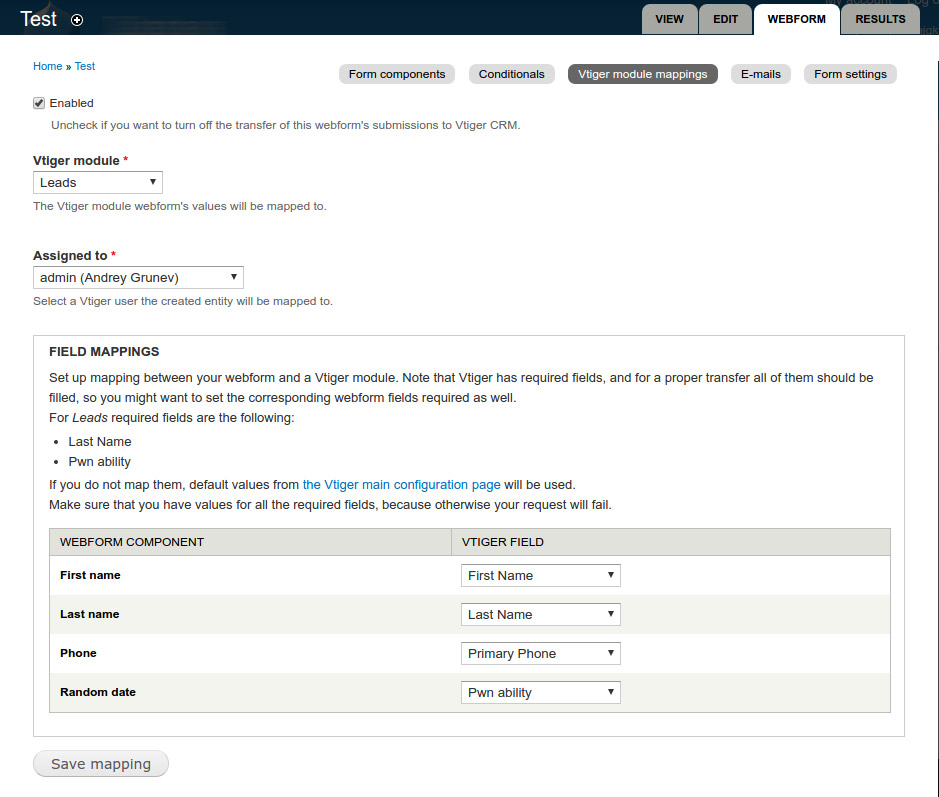The image showcases a detailed view of a "Vtiger Module Mappings" page within a computer website form interface.

At the top, a black banner with the word "test" in white letters is displayed alongside a white circle containing a plus symbol. Below, there are three tabs: "View" and "Edit" in black text on gray tabs, and "Results." The currently selected tab, "Web Form," is highlighted. Breadcrumb navigation shows "Home" followed by an arrow pointing to "test" in blue.

Action buttons under the banner include "Form Components," "Conditionals," "Vtiger Module Mappings," "Emails," and "Form Settings." The selection "Vtiger Module Mappings" is blacked out, indicating it's currently active. A check mark next to "Enabled" denotes its active status, with an option to uncheck for disabling the transfer of this web form's submission to the Vtiger CRM.

The form includes a dropdown menu labeled "Vtiger Module" with "Leads" selected. This module's web form entries will be mapped to specified fields within Vtiger. Another section titled "Assigned To" features a dropdown with "Admin Andre Grunev" selected, designating the Vtiger user to whom the created entity will be assigned.

Further down, the "Field Mappings" section guides users to align web form data with Vtiger module fields, emphasizing the need to fill all required fields to avoid transfer errors. For the "Leads" module, the required fields listed include "Last Name" and "PWN Ability." If these fields are not mapped, default values from the Vtiger main configuration page will be used.

The form fields displayed on a gray background include:

1. "First Name" with a rectangular input box and dropdown arrow.
2. "Last Name" in bold black text followed by another rectangular input box.
3. "Phone" in bold black text with "Primary Phone" in a rectangular input box.
4. "Random Date" on a slightly gray background with "PWN Ability" in a rectangular input box and dropdown arrow.

A button labeled "Save Mapping" appears at the bottom, concluding the form.